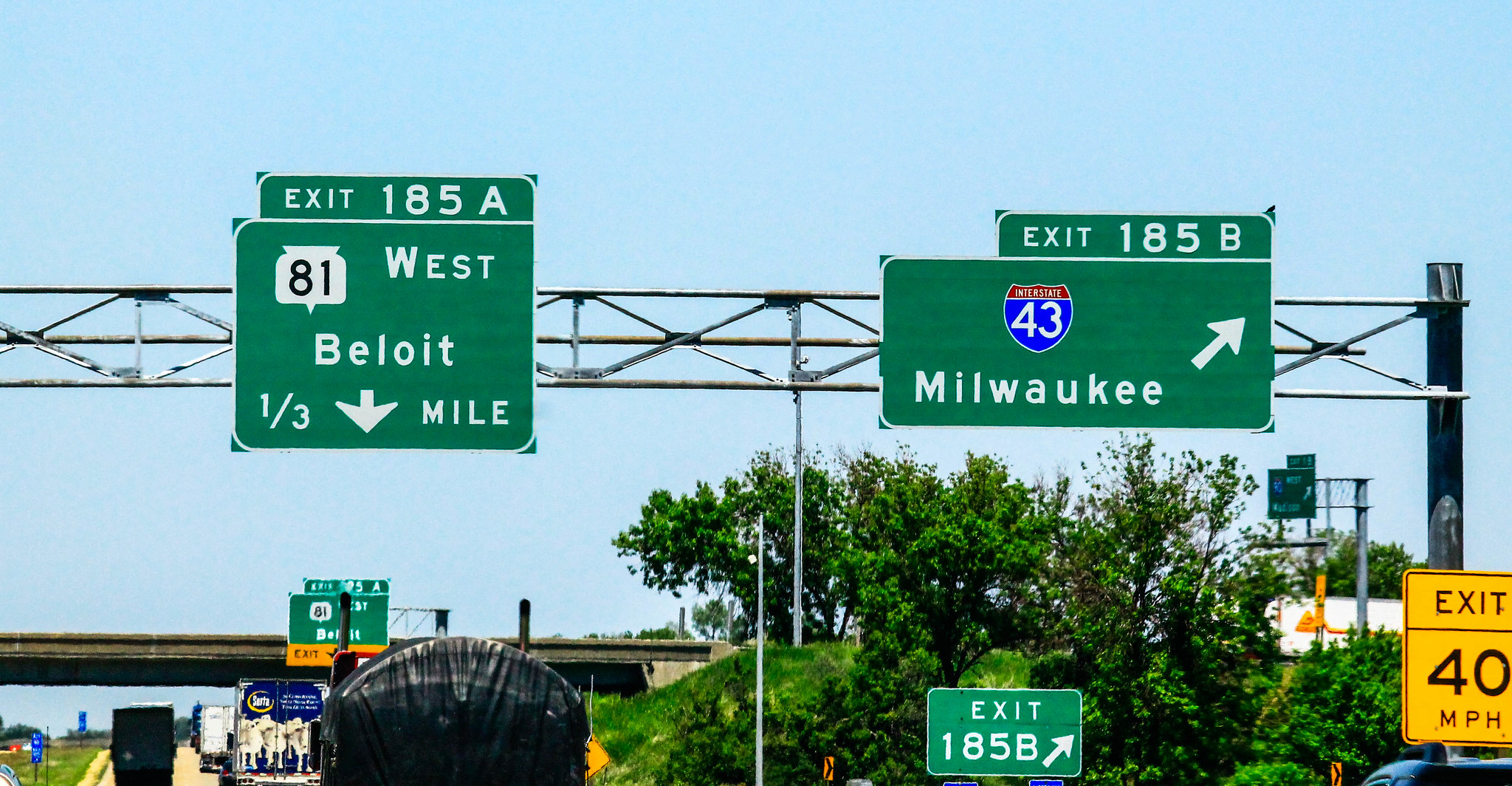This image depicts a scene from a highway near Milwaukee with clear signage for drivers. Prominently featured overhead are two green interstate signs guiding traffic for upcoming exits. On the right, the first green sign indicates Exit 185B, displaying the red and blue interstate shield with '43' labeled on it and an arrow pointing right towards Milwaukee. To the left, another green sign for Exit 185A instructs drivers with a downward arrow to stay in their lane. It reads '81 West Beloit' spelled out as B-E-L-O-I-T, and mentions the distance of one-third mile. Below these main signs, in the bottom right corner of the image, a gold sign warns drivers to reduce their speed to 'Exit 40 MPH'. Additionally, on the left-hand side, several tractor-trailers can be seen traveling down the road below the signage. There is also some foliage and a couple of trees in the vicinity, adding a touch of greenery and splitting the paths of the two exits.